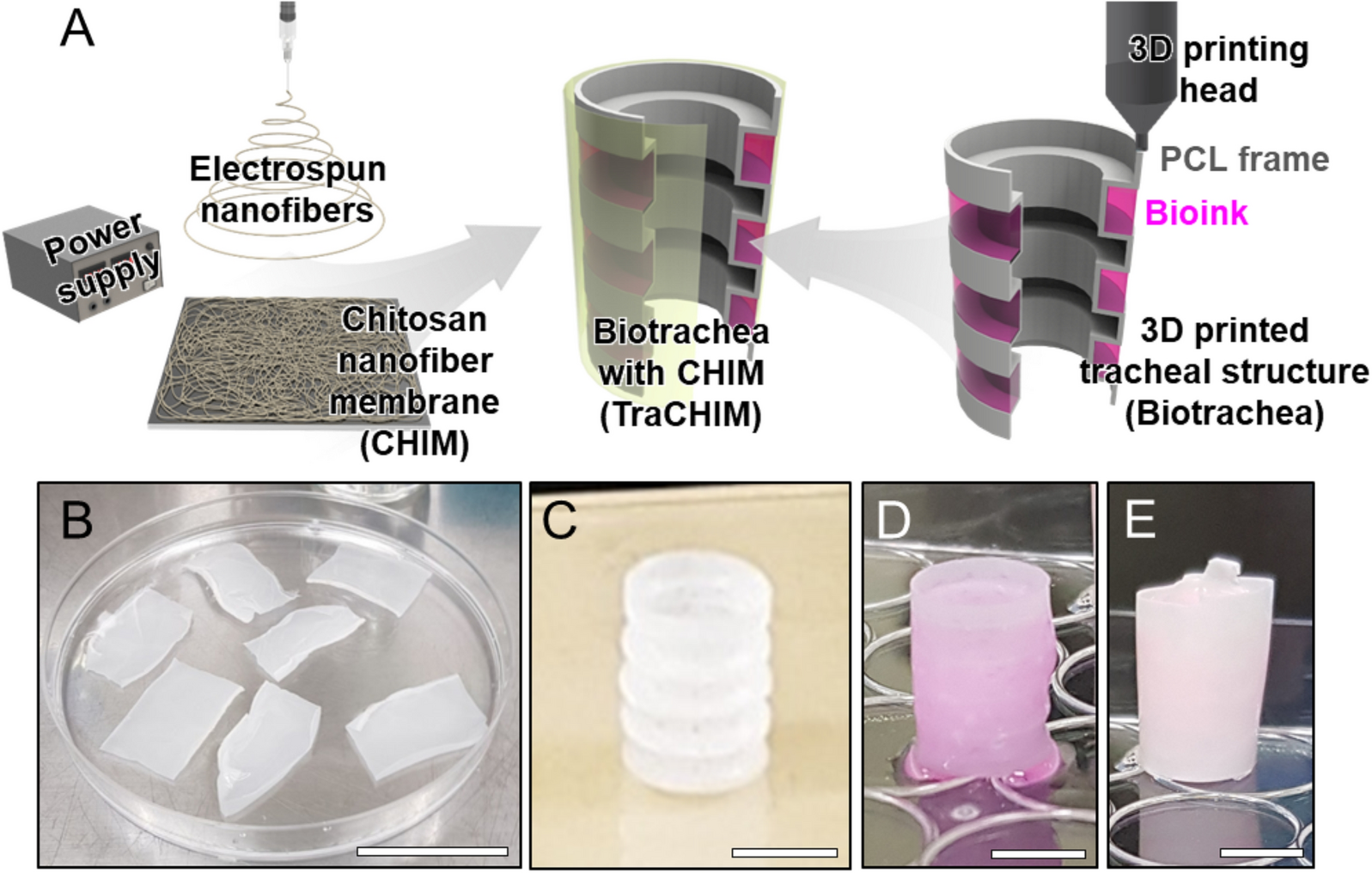The image displays a detailed scientific diagram at the top, labeled A, illustrating a 3D printing process involving various materials and components. From left to right, the labels describe a power supply depicted as a gray box with buttons, electrospun nanofibers represented by a coil, a chitosan nanofiber membrane shown as a square piece, and biotrachea with "CHIM." The biotrachea is displayed as a half-cylinder structure. An additional label points to a 3D print head, PCL frame, and bio-ink, which is pink, culminating in a 3D printed tracheal structure. Below the diagram are four photographs labeled B, C, D, and E. Photograph B shows a petri dish containing small sheets of plastic or glass. Image C features a white cylindrical object, which appears coiled. D depicts a similar cylindrical object in pink, suggesting a waxy texture. Lastly, E presents another white cylinder with a smooth surface, resembling a crystal. Together, these elements illustrate the stages and materials involved in creating a biotracheal structure using 3D printing technology.